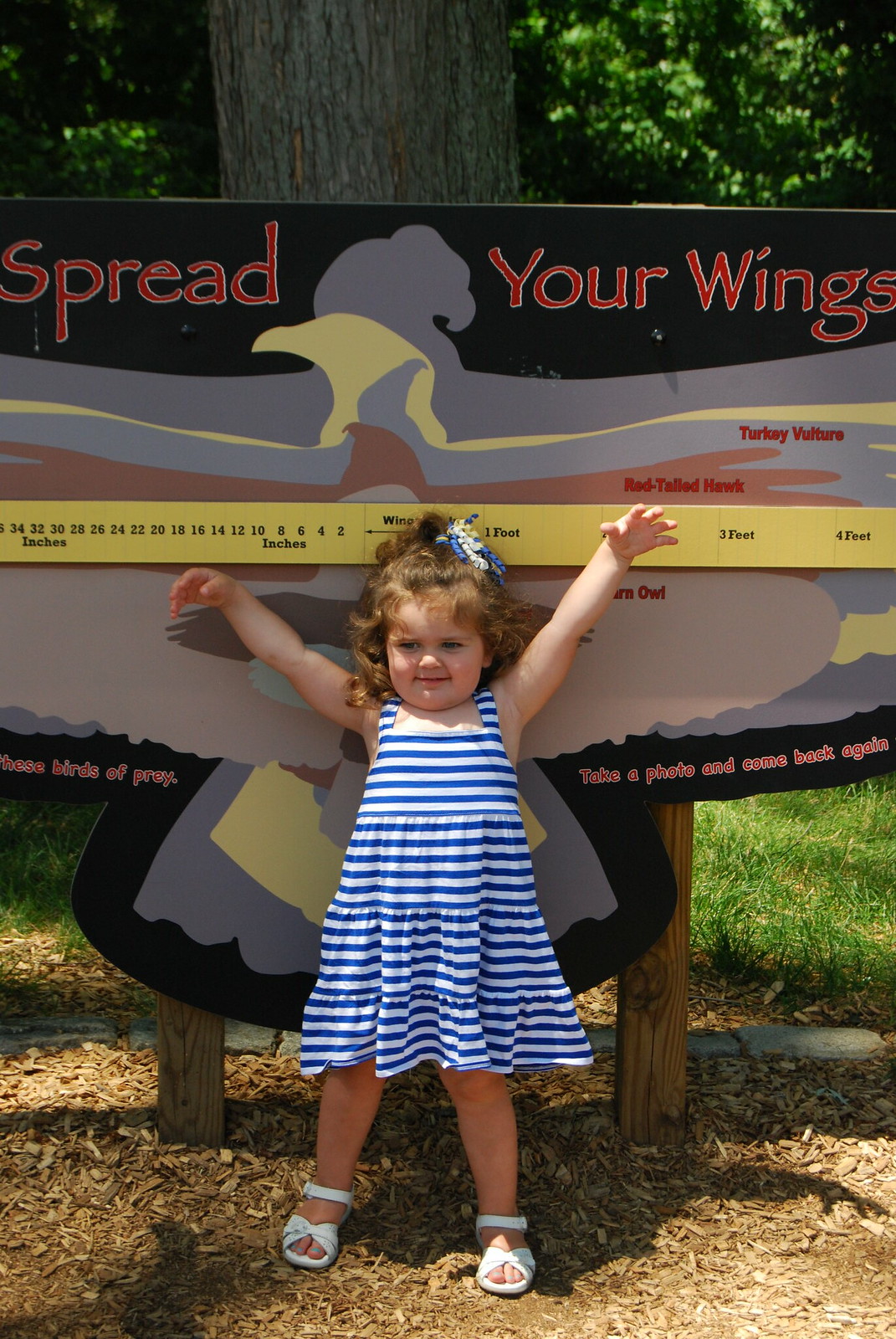In this vibrant, full-color photograph taken outdoors on a sunny day, a young white girl stands out as the central figure. She is around three years old, with curly light brown hair adorned with a blue and white ribbon that trails through her locks, resembling more of a ribbon than a bow. The little girl is dressed in a charming knee-length sundress featuring navy blue and white stripes, paired with delicate white sandals. Her arms are outstretched wide, almost like wings, as she strikes a playful pose.

Behind her, a whimsical scene unfolds. A tree trunk with lush green leaves frames the setting, and the ground underfoot is a mix of brown dirt and patches of green grass. A prominently placed sign in the background, with bright red letters reading "Spread Your Wings," features the drawing of a bird, possibly a turkey, with wings fully extended. This sign doubles as a measuring stick, illustrating the stretch of the girl's arms, which reach an impressive 20 inches. The image is captured with a funhouse mirror-like effect, giving it a quirky, slightly distorted appearance that adds an extra layer of delight to an already heartwarming scene.